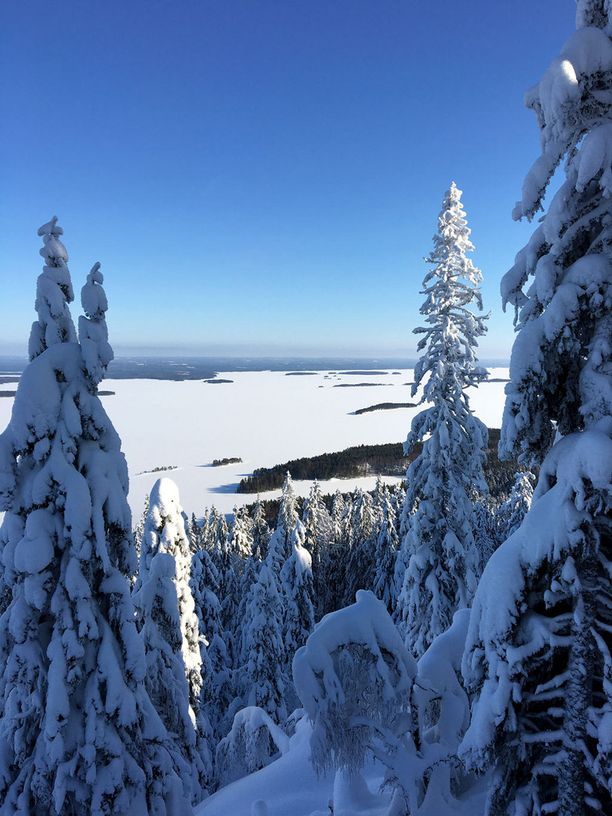The photograph, captured in portrait orientation, showcases a stunning snowscape dominated by evergreens heavily laden with thick, wet snow. The dense branches, weighed down by the accumulation, arc gracefully towards the ground, providing a natural frame for the image. Along the bottom of the frame and extending up the right-hand side, these snow-covered evergreens create a picturesque border. 

The vantage point suggests the photographer is positioned on the slope of a mountain or hill, offering a sweeping view of an expansive, snow-covered landscape that extends to the horizon. Dozens of similarly snow-cloaked trees populate the scene, highlighting the aftermath of a substantial snowfall. This was no light flurry; it was a significant snowstorm, which left a velvety blanket of snow over every visible surface. 

Beyond the immediate foreground, the terrain opens up. While the precise nature of the vast expanse is unclear—it could be a frozen waterway, a large field, or a meadow—it is entirely enveloped in white. A few small rows of trees punctuate the snowy vastness before it stretches endlessly into the distance. The day itself is pleasantly clear, with a bright blue sky overhead and no clouds in sight, indicating that the heavy snowstorm had passed, leaving behind this serene, winter wonderland.